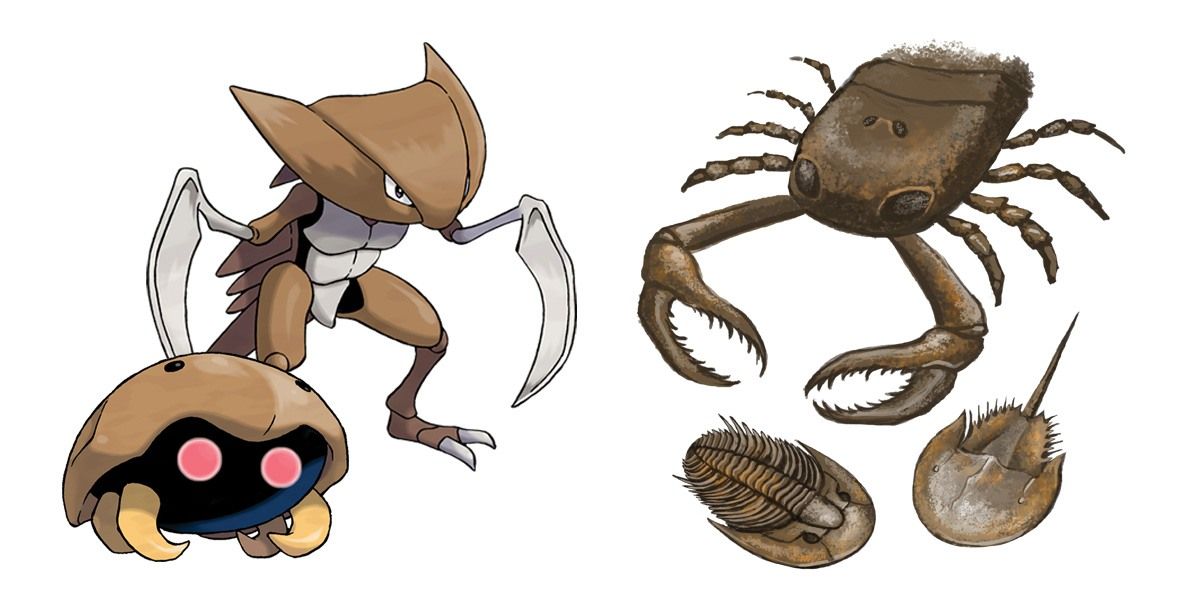The image depicts a blend of animated and realistic creature designs inspired by various types of bugs and marine animals. On the left side, there is a small, animated beetle-like creature with a hard, brown shell, glowing red eyes, and four legs. Above it stands a larger animated figure with a brown head, a white torso, and two drooping blade-like arms, resembling a dinosaur-insect hybrid. On the right side, a sequence of more realistic, crab-like creatures is shown. One notable figure has a circular, brown body with eight legs and strong pincers. It has two large brown eyes and is accompanied by smaller, flat brown creatures with sharp protrusions. The design elements blend features of trilobites and horseshoe crabs, with a distinctly alien appearance, merging natural and fantastical elements seamlessly.